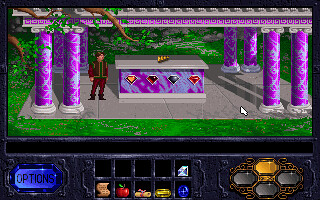This image is a screen capture from a video game, presented in a wide, horizontally rectangular format. The upper two-thirds of the screen displays the game environment, while the lower third contains various user interface elements. The top section illustrates a lush, green grassy area flanked by four imposing purple pillars located at each corner: bottom left, bottom right, top left, and top right. These pillars support a gray stone platform that spans horizontally across the scene.

In the central area of the grassy expanse is a concrete patio featuring a large, ornate altar or casket. The casket has a gray top and purple sides adorned with four colorful diamond-shaped gems. From left to right, the first gem is yellow, followed by a red gem, a blue gem, another red gem, and another blue gem. Standing to the left of the casket is a character dressed in a brown shirt and brown pants with short brown hair, facing the altar.

The lower third of the screen contains the game's user interface, which is gray and divided into several sections. On the far left, there is a blue button resembling a sapphire, labeled "Options." To the right of the Options button, there are two rows of black cubbies in a 5x2 grid, where various collected items such as gemstones, an apple, and a scroll are displayed. In the bottom-right corner of the interface, there is a circle adorned with squiggly designs, containing four icons or rubies. The upper left ruby is lit up in orange, indicating an active or selected state.